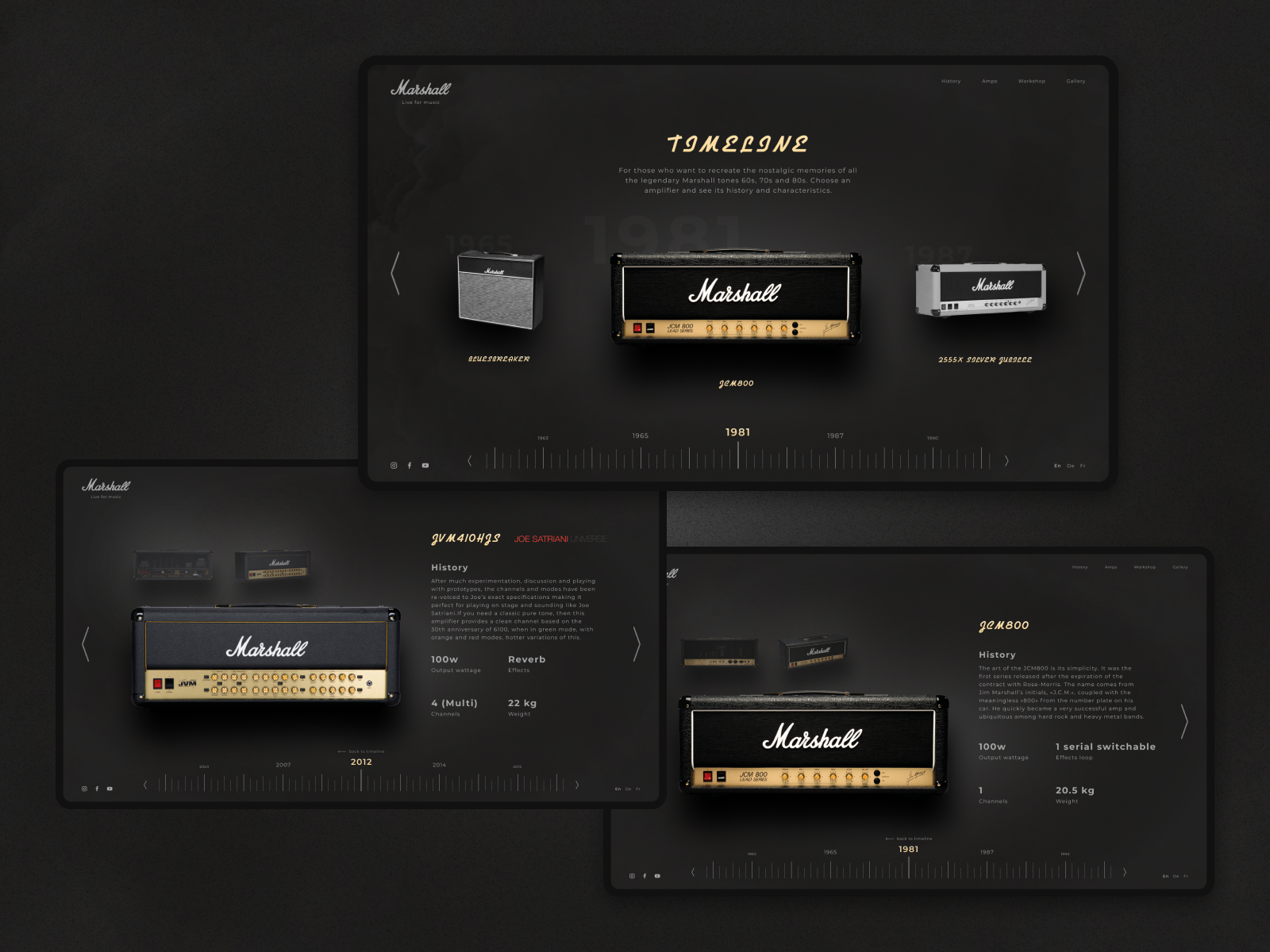This detailed caption describes the image:

"Depicted in the image is a recreated version of a classic Marshall amplifier. The top right corner of the image features text, which begins with the letter 'T', though the full word is unclear. This amplifier is the result of extensive experimentation, discussion, and the development of numerous prototypes. It offers multiple channels and modes identified as 'THO' and '6X', enhancing its sophistication and making it ideal for live stage performances. 

The design includes a notable reverb feature, adding a formal tone to its sound. The amplifier is marked with 'SEM 1981', indicating its model possibly related to the iconic JCM800 series known for its simplicity and rapid adoption by users. One notable switch on the amplifier allows for channel selection, and the whole unit weighs approximately 20.5 kilograms. The amplifier's exterior features a grey color scheme, and the overall image suggests it is a piece of sophisticated machinery designed for quality sound delivery."